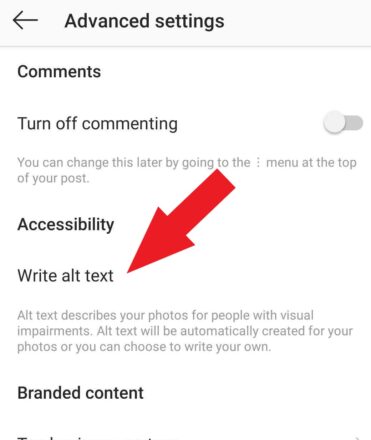At the top of the image, a gray section features a left-pointing black arrow and the words "Advanced Settings." Below this area, set against a white background, the word "Comments" is prominently displayed. Directly underneath, an option labeled "Turn Off Commenting" is accompanied by a gray toggle bar currently set to the left. 

A line of text follows, stating, "You can change this later by going to the ellipsis menu at the top of your post." Moving down, the word "Accessibility" is present, followed by another line of text that reads "Write Alt Text," highlighted by a large, red, downward-pointing arrow. 

Further down, the section continues with a description under "Alt Text," explaining: "Alt text describes your photos for people with visual impairments. Alt text will be automatically created for your photos, or you can choose to write your own." Beneath this, a new section titled "Branded Content" appears in black text, followed by a series of four black dots aligned in a line.